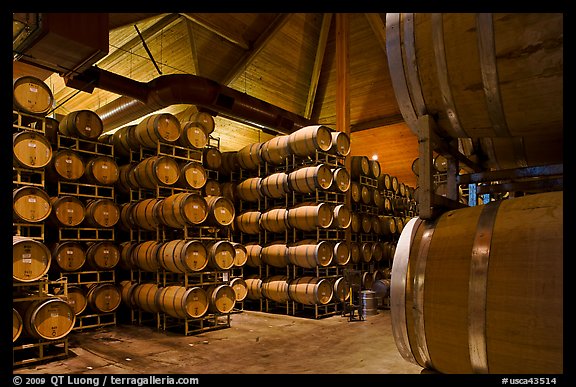This image depicts the interior of a winery’s barrel storage area, showcasing rows upon rows of large wooden casks and barrels stacked up to five high on sturdy metal racks. The high, cathedral-like ceiling adds to the grandeur of the scene, featuring exposed vent pipes that enhance the industrial ambiance of the space. The architectural design marries wood and metal elements beautifully, creating an aesthetically pleasing and functional storage environment. The floor appears to be utilitarian, made of a material neither extravagant like tile nor purely wooden, ensuring practicality for the area. In the bottom left corner, the photo is marked with a copyright date of 2009 by QT Luong, and it directs to terragalleria.com, indicating the photographer's work.